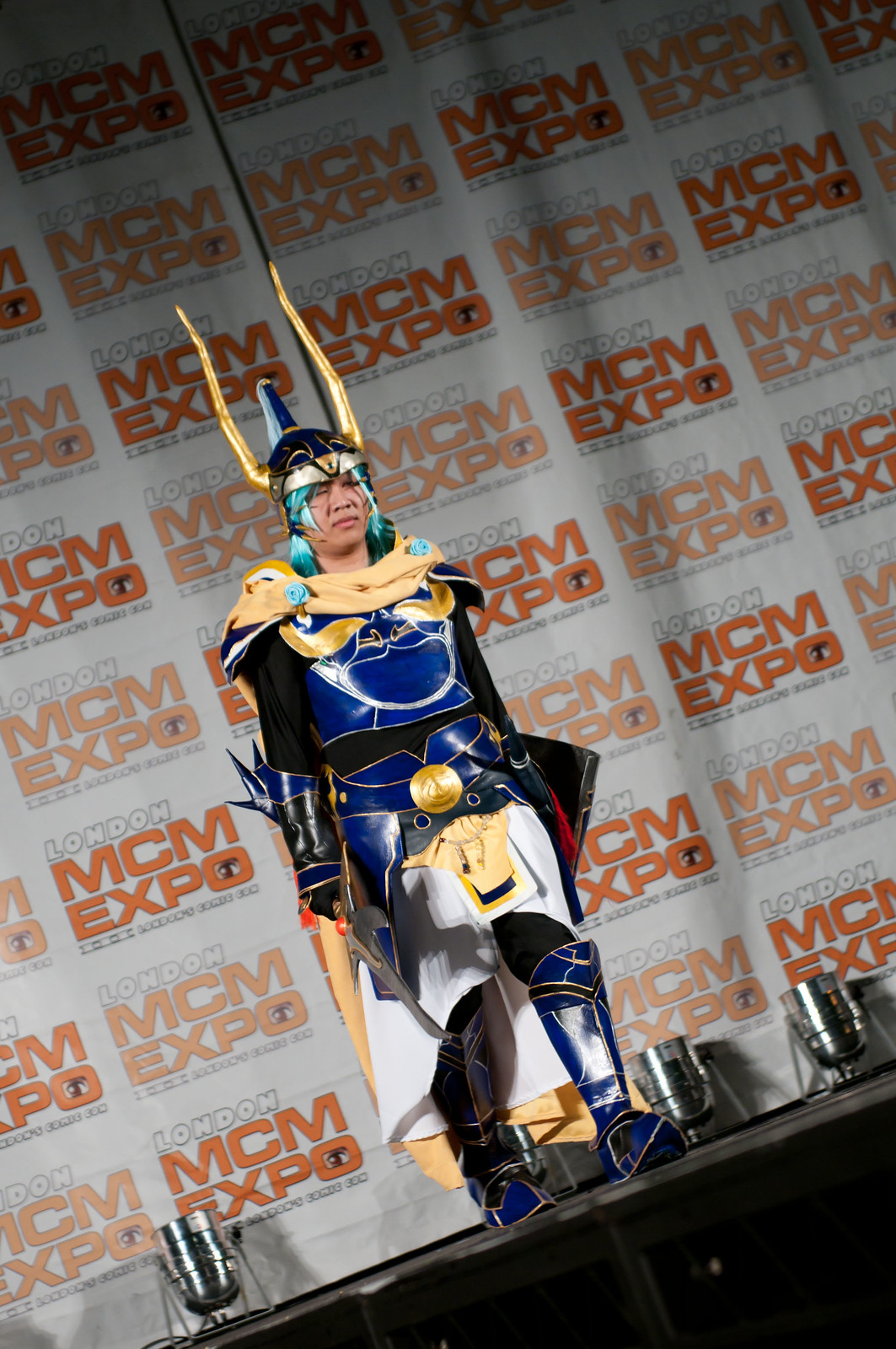In this slightly tilted photograph of an indoor stage at the London MCM Expo, a person dressed in an elaborate costume stands prominently on a black stage. The costume features a striking mix of blue, gold, and white. The individual wears a blue helmet adorned with long, straight golden horns protruding upwards, reminiscent of Viking or Egyptian headgear. Below the helmet, the person has light blue and white-dyed hair or a wig.

The upper body of the costume includes blue and golden armor, complemented by a yellow robe draped over the shoulders. The belt is also blue and gold, adding to the ensemble's superhero-like appearance. The lower body is adorned with a white skirt typical of a warrior’s garb, blue and yellow boots, and black leggings. Arm guards with blue spikes contribute to the overall warrior aesthetic. The individual holds a sword, presumably a prop, in one hand.

Behind the figure, the stage is equipped with silver-colored lights, and a large white poster with the recurring orange text "London MCM Expo" fills the background, contextualizing the event as a comic-con-like gathering.